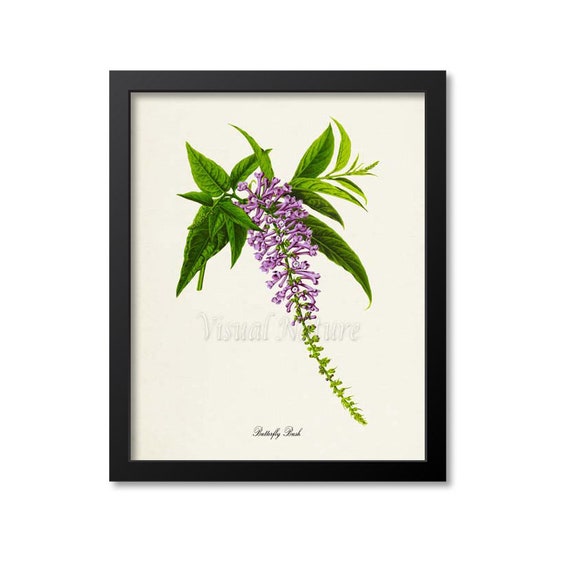The image depicts a matted and framed botanical-style photograph with a watermark that reads "visual nature." The artwork is enclosed in a basic black frame with a white matting and a cream-colored background, designed to be sold as decorative wall art. The focal point of the photograph is a unique flower that closely resembles the shape of an elephant's trunk and showcases a gradient of colors, starting with a vibrant lilac purple at the top that narrows down into a green stem with small branches and leaves. The flower emanates from a spray of teardrop-shaped, green leaves at the top. There is also a legend at the bottom of the image that partially reads "butterfly," possibly indicating the name "butterfly pea." The photo includes some illegible cursive text, likely identifying the artist or the piece.